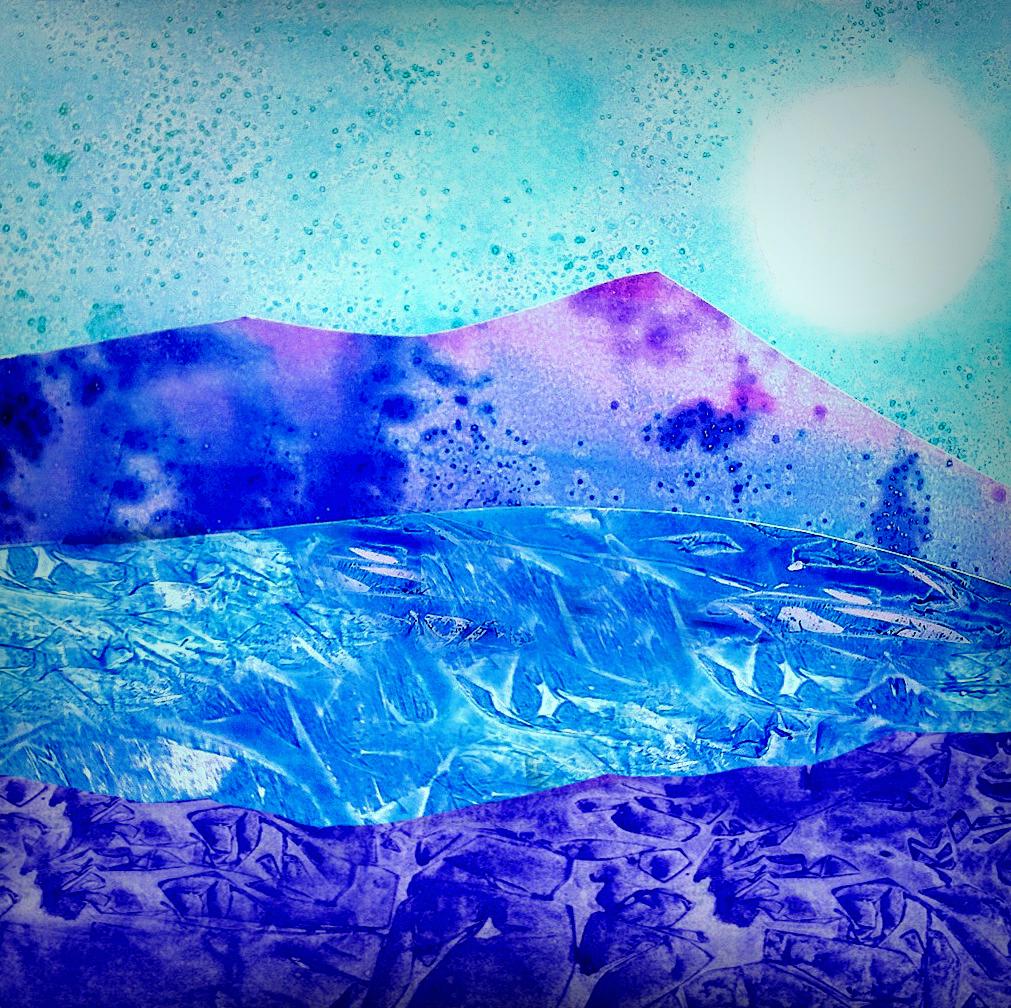The image presents a vibrant and abstract interpretation of a landscape, dominated by a color palette of dark blues, purples, light blues, and whites. In the top right corner, a bright, circular sun stands out against the sky, which is a blend of light blue and white, with small, darker blue splotches resembling paint splatters or raindrops on a window. Below the sky, the scene transitions into a mountainous region, characterized by a chaotic but visually captivating application of blue and purple paints, seemingly splashed and mixed together giving it an impressionistic feel. The landscape continues with what appears to be a serene, icy-blue lake, reflective and evocative of cold water. At the very bottom, a land area painted in dark blue hues, marked by indistinct shapes suggesting grass or terrain, completes the layered composition. The deliberate and artistic use of color creates a cohesive and striking visual theme, devoid of any text, that captures the viewer's imagination with its abstract beauty.